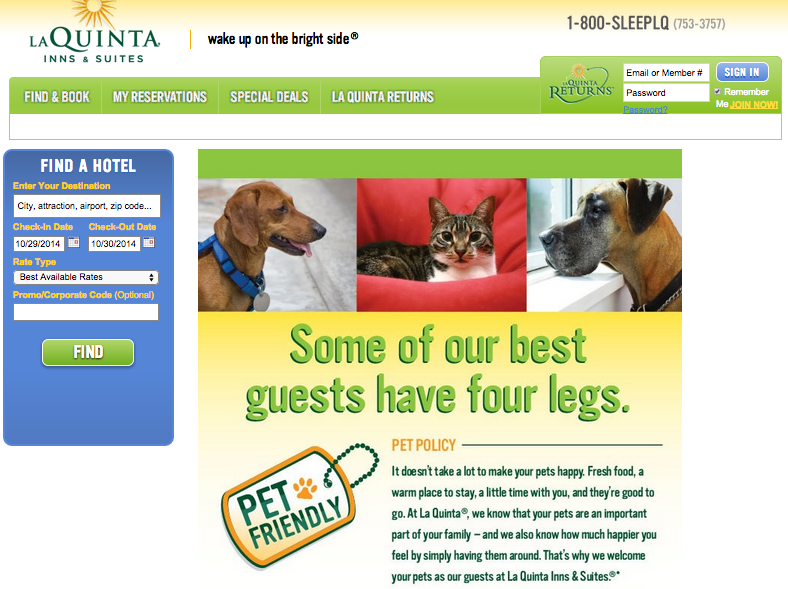Here is a detailed and cleaned-up caption for the image:

---

This image is an advertisement for La Quinta Inns and Suites. The top portion features a color gradient of yellowish and white hues, with a sun symbol prominently displayed in the top left corner. The brand name "La Quinta Inns and Suites" is written in green across the upper part of the image. To the right of the logo, there is a 1-800 number that reads "SLEEPLQ." 

In the upper right section, the text "WAKE UP" is visible next to the sun symbol. Below the main logo, there is a navigation bar with tabs labeled "FIND AND BOOK," "MY RESERVATIONS," "SPECIAL DEALS," and "LA QUINTA RETURNS." To the far right of this navigation bar, there is a section for La Quinta Returns members, prompting users to enter their EMAIL or MEMBER NUMBER in the top box and their PASSWORD in the bottom box. Below these fields are the options to "SIGN IN," check "REMEMBER ME," and a "JOIN NOW" button.

On the left side, within a blue box, is a "FIND HOTEL" button. The lower center part of the image features the text "SOME OF OUR BEST GUESTS HAVE FOUR LEGS," accompanied by a dog tag labeled "PET FRIENDLY." To the right of this is the "PET POLICY" link.

---

This enhanced caption provides a detailed and structured description of the image, making it easier to understand the various elements and their placements.